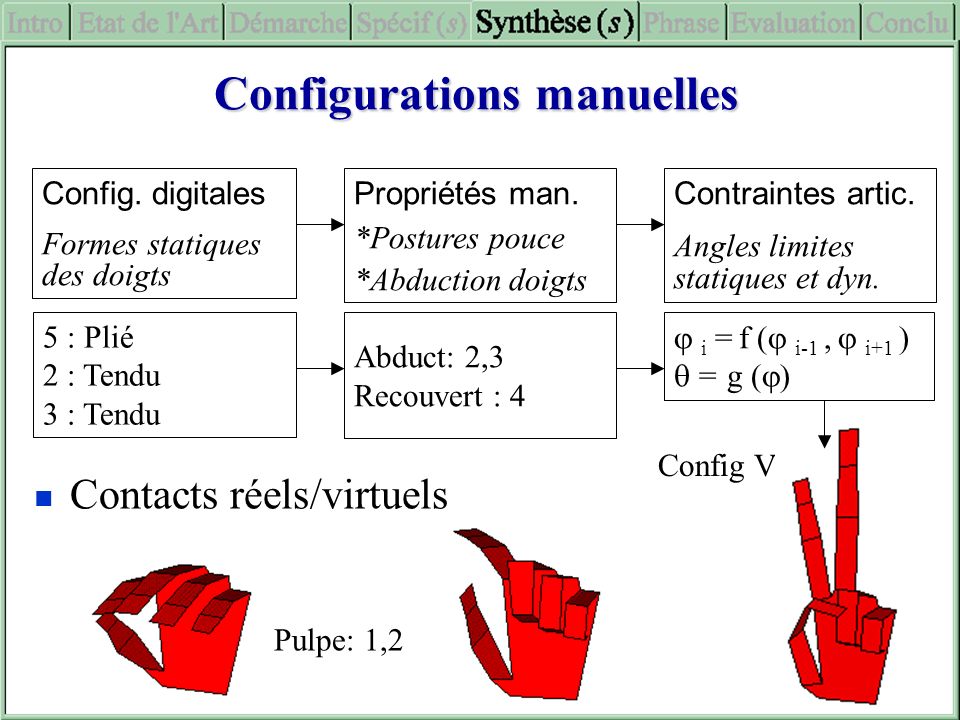This image is an informational diagram written in French, describing different hand configurations. At the top of the infographic, there is a title labeled "Synthès Parentheses S" followed by several sub-headers and text boxes that outline various configurations and properties, including mathematical symbols and annotations. The text uses both blue and black fonts for different sections. The bottom part of the infographic features three red, paper-like drawings of hands in different positions: one with the thumb touching the index finger with the other fingers bent, another with the thumb and index finger extended while the other fingers are curled down, and a third with the index and middle fingers extended upwards like a peace sign, with the thumb curled upwards. These images seem to illustrate configurations or postures for some kind of study or manual.